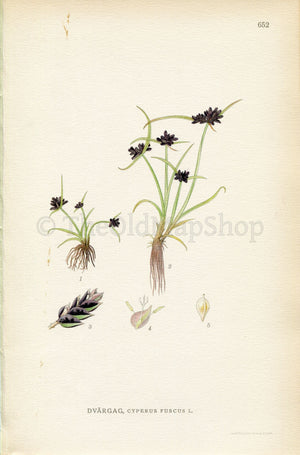The image is a vertically aligned rectangle, resembling an older book page. In the upper right-hand corner, the page is marked with the number 652 in gray. A prominent watermark across the center reads "The Old Map Shop" with each word capitalized. The page itself appears yellowed with visible brown stains and wrinkling, particularly on the left side.

Central to the image are detailed botanical illustrations. These include multiple plants with green stems, some of which have been uprooted, displaying their brownish roots. The plants feature black and purple or black petals, as well as blooming flowers on some stems. There is an arrangement of leaves that are white on the outer edges with black interiors. Additionally, the lower portion of the image depicts various smaller drawings, including a teardrop-shaped object and a seashell-like shape pointing downward. The Latin names of the plants are inscribed at the bottom, though they are difficult to decipher due to their small size.

Overall, the depiction is both intricate and colorful, set against a predominantly white background, capturing the essence of vintage botanical artwork.